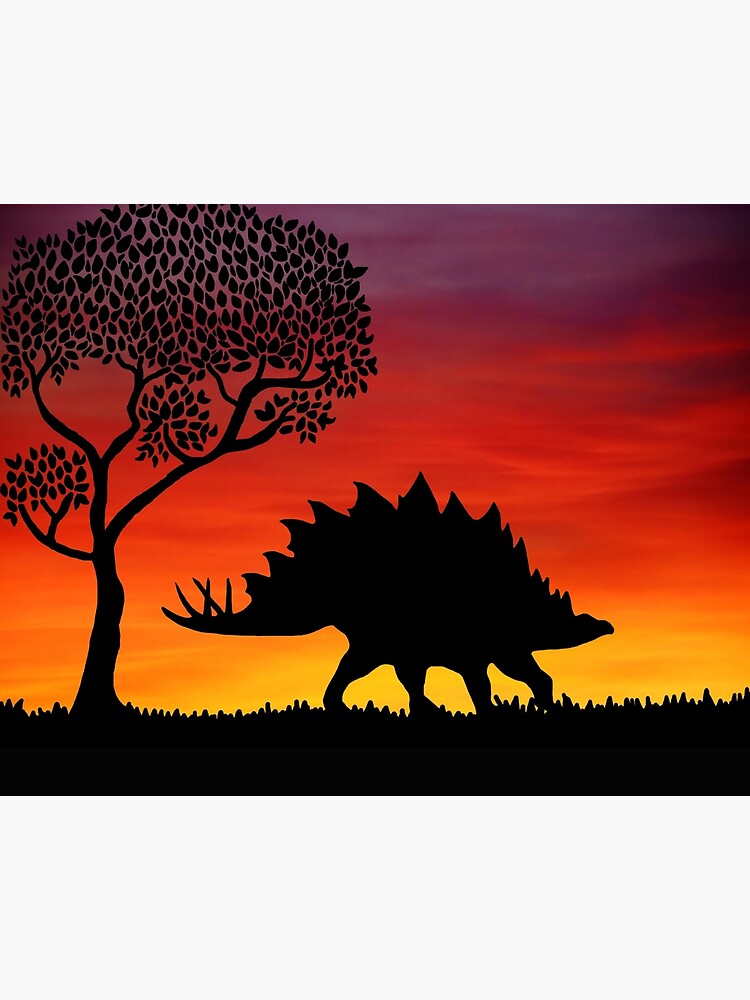A dramatic, silhouetted scene features a Stegosaurus walking on a black, grassy ground during a breathtaking sunset. The Stegosaurus, visible in profile with signature plate spikes along its spine and longer, thinner spikes on its tail, heads toward the right. To its left stands a stylized tree with several branches adorned with detailed leaves. The sky behind them is a vibrant tapestry of colors, transitioning from bright yellows and oranges at the horizon to deep reds and purples higher up, reminiscent of a watercolor painting. This vivid sunset casts the prehistoric landscape in striking contrast, enhancing the dramatic and timeless feel of the image.